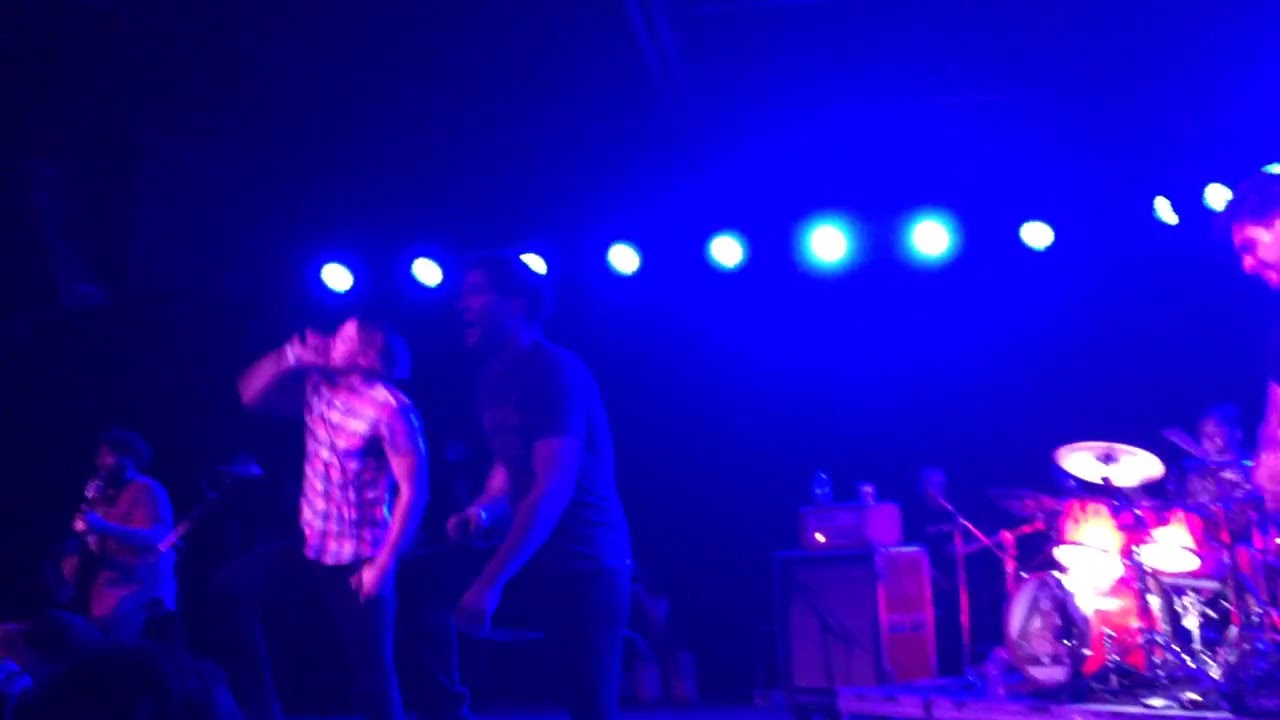The photograph captures a vibrant scene inside a music club bathed in intricate blue and white lighting. At the center of the stage, a band performs energetically. You can see a drummer behind a well-lit drum set, vigorously playing. To the side, another musician, clad in black jeans and a short-sleeved shirt, sings passionately into a microphone, engaging with the crowd. In the blurred background, a man in a plaid shirt also sings into a microphone. A guitarist with longish hair adds to the ensemble's dynamic performance. Scattered around the stage are essential equipment pieces, including amplifiers with water bottles resting on top, and numerous microphones set up for the performance. The overall atmosphere is dimly lit aside from the prominent blue light that bathes the venue, highlighting the intense and immersive concert experience for both the band and the audience.